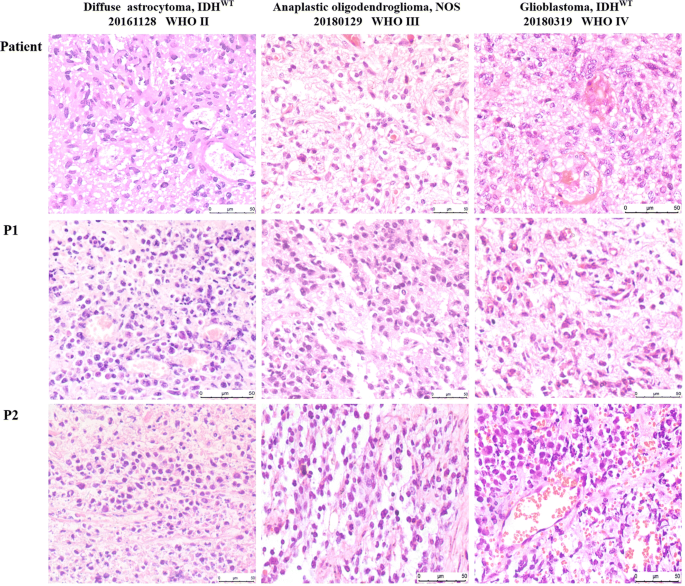The image is a large, square, composite figure consisting of nine smaller, square, microscopic images arranged in a 3x3 grid, each separated by a white line. Each row and column in the grid is labeled, with the columns headed by different types of brain tumors: "Diffuse Astrocytoma IDH 2016128 WHO II," "Anaplastic Oligodendroglioma NOS 20180129 WHO III," and "Glioblastoma IDH 20180319 WHO IV." The rows are labeled from top to bottom as "Patient," "P1," and "P2."

Each of the nine squares displays a micrograph of cells, primarily showcasing shades of purple, with some specks of darker purple and hints of white and pink. These are likely representations of various brain cancer cells, potentially highlighting different patients' samples. The visual texture within the squares consists of swirls and dots of purple, varying in pattern without any obvious order. A small, unreadable scale appears on each image, indicating the magnification level of the microscopic views.